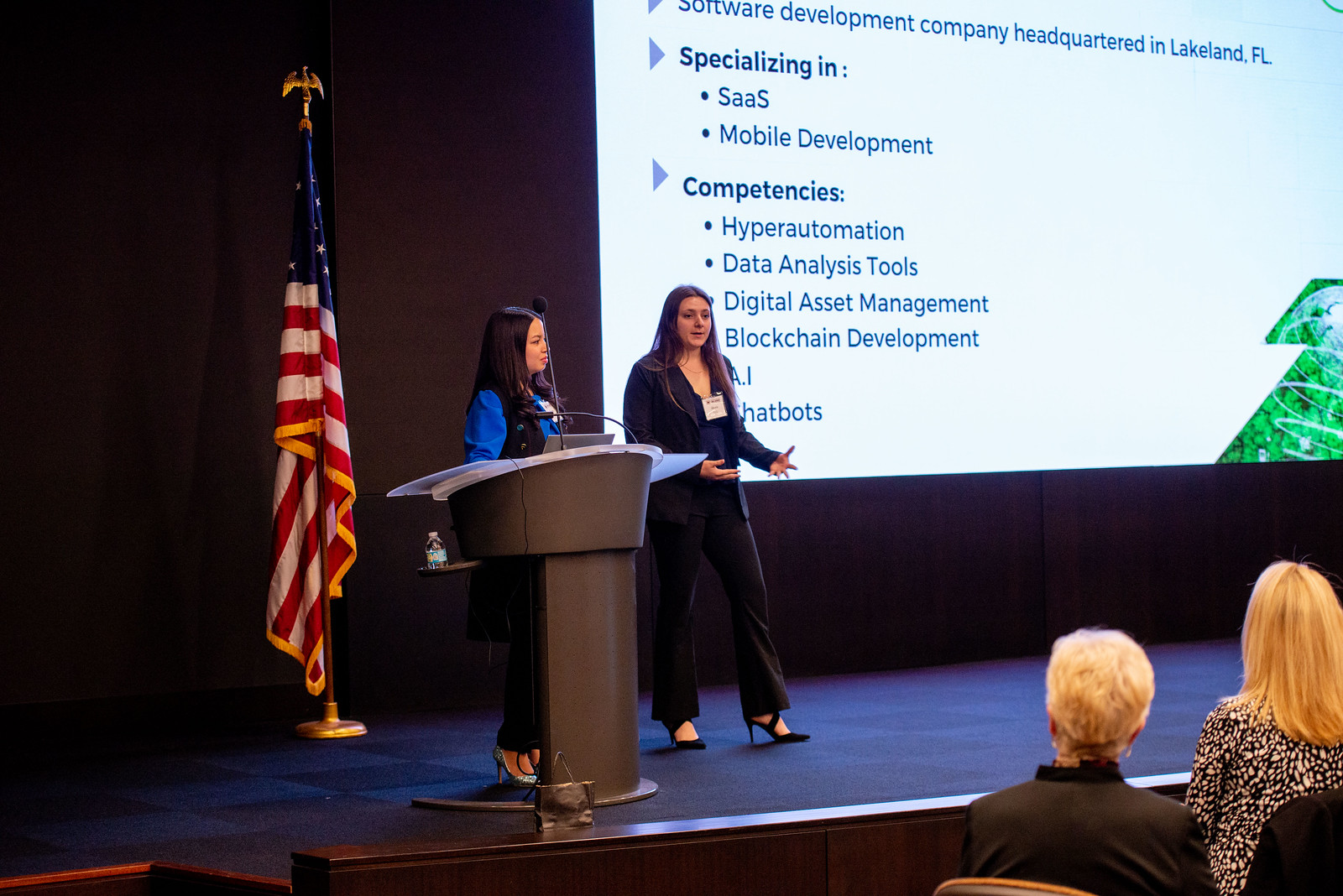The photograph captures a scene from a presentation or conference event featuring two women on stage. The woman on the left, standing behind a gray podium equipped with a microphone, has long dark hair and is dressed in a blue top, black pants, and high-heeled shoes. To her right stands another woman with a long business jacket, black pants, and high heels. She has a name badge draped around her neck, reaching down to her chest, and she is gesturing with her hands as she speaks, slightly facing forward and to the left. Both women have dark, long hair. An American flag on a gold stand is positioned to the left of the women, while a large screen forms the backdrop of the stage. The visible text on the screen appears to have a white background with black text detailing the services of a software development company headquartered in Lakeland, Florida. The text mentions specialties such as SAAS, mobile development, hyperautomation, data analysis tools, digital asset management, blockchain development, AI, and chatbots. Additionally, a bottle of water is placed on the podium. In the bottom right corner of the image, partially visible, are two audience members seated in chairs with their backs to the camera. The audience member on the left has short blonde hair and is dressed in a dark top, while the one on the right has longer blonde hair and wears a black and white top. The stage is covered with blue square carpeting, adding a formal touch to the setting.